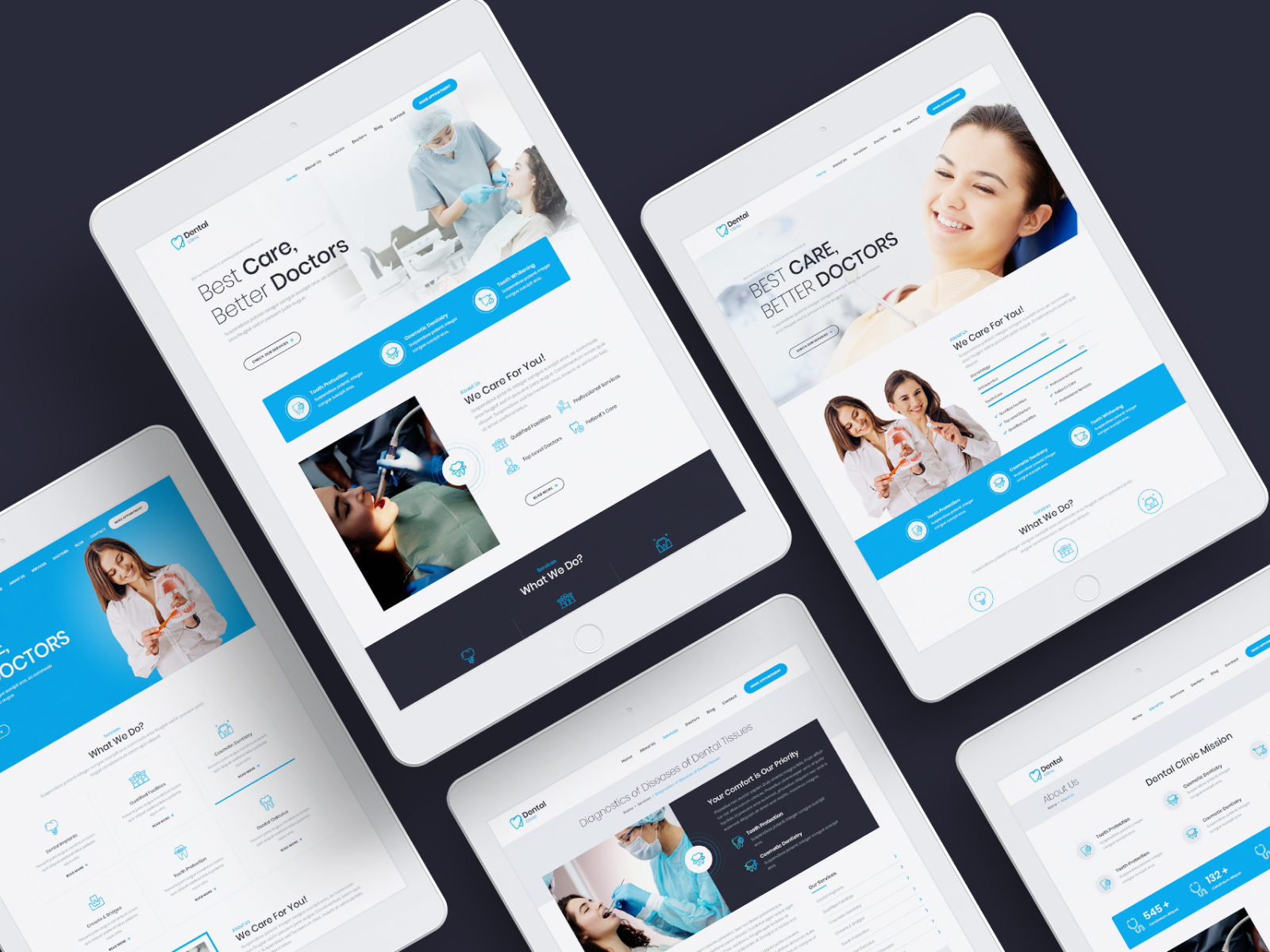The image features five white iPads, prominently displaying advertisements related to dental care and doctor services. Out of the five iPads, only two are fully visible. Each iPad showcases images and text promoting better healthcare and better doctors, with a specific focus on dental care. The background of the image is a dark blue, almost black, providing a stark contrast to the white iPads.

The advertisements feature several individuals who appear to be either White or Asian. These individuals are depicted either holding dental devices, such as toothbrushes, or reclining in dental chairs. There are also two dental professionals, identifiable by their head coverings and surgical masks, attending to the patients' dental needs.

The ads emphasize the theme of superior care through slogans like "better care, better doctors," and include informational sections titled "what we do." Each iPad screen offers several hyperlinks, suggesting additional resources or further information. The scene is devoid of any other notable features or objects, keeping the focus solely on the iPads and their displayed content.